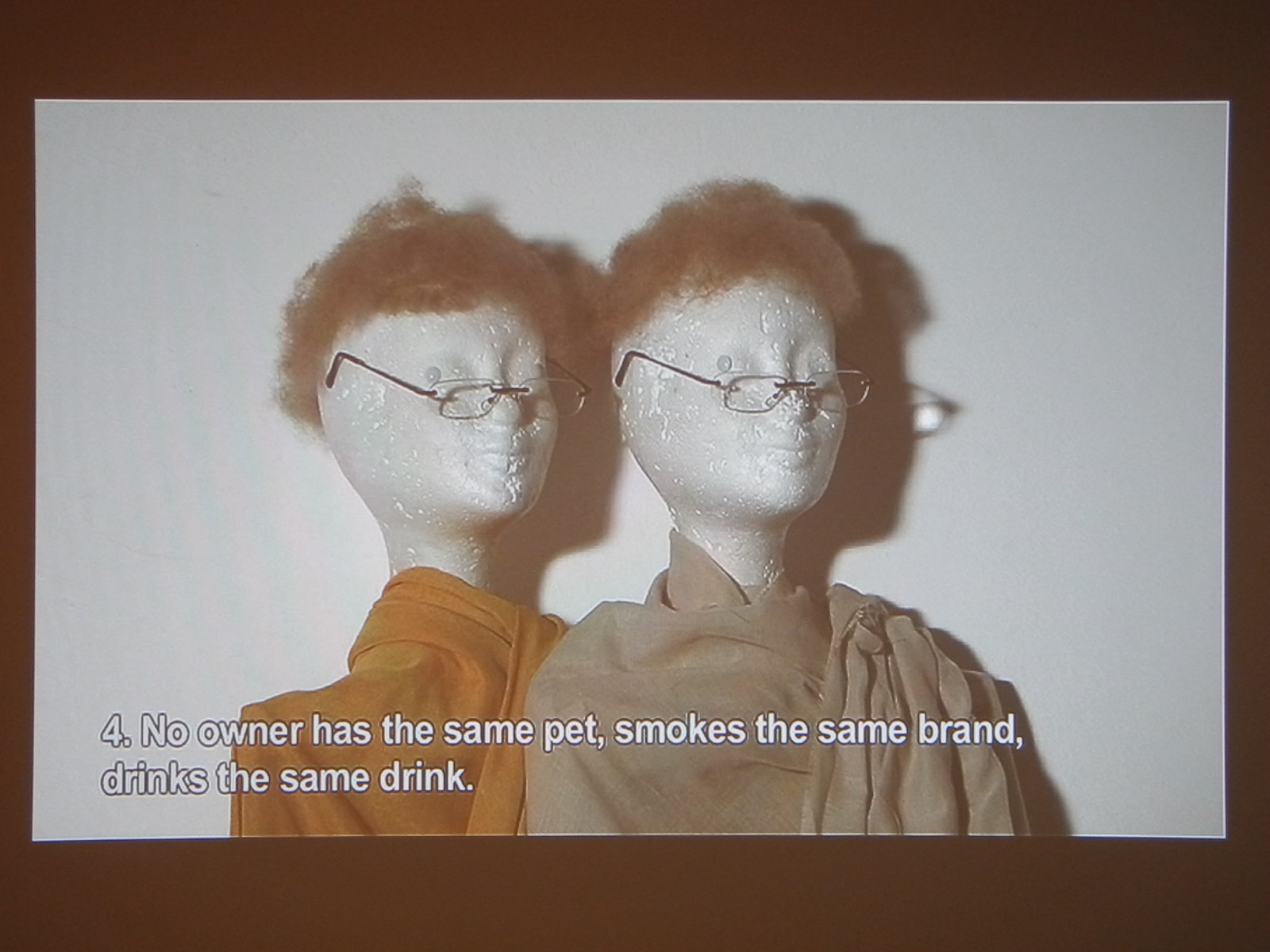A detailed photograph depicts two styrofoam mannequins standing side by side in front of a stark white wall. Each mannequin sports a fuzzy blonde wig and chic sunglasses. Their surfaces are textured with numerous small divots, giving them an intricate yet simple appearance. The mannequins are draped in blankets; one enveloped in a vibrant orange blanket, while the other is swathed in a soft light gray one. Shadows cascade behind them, cast upon the wall by a light source. At the bottom left of the image, a poignant message appears in white font, reading: "for no owner has the same pet, smokes the same brand, drinks the same drink."